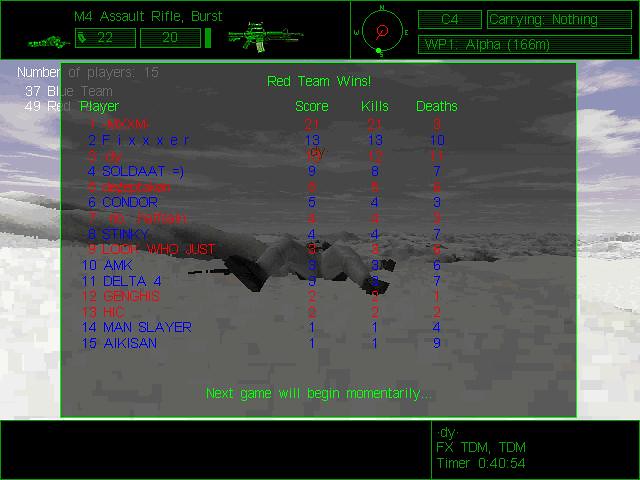In this color image from a video game, the victorious screen displays the aftermath of a round. Dominating the center panel, which is outlined in green, is a black and white image of a pixelated character lying down, signifying defeat. At the top, bold text proclaims "Red Team Wins" in a striking font. 

The left side of the panel features a list of players, arranged from top to bottom, each accompanied by their corresponding scores, kills, and deaths, which are highlighted in red and blue colors to differentiate the teams. Beneath this panel, a green text announces, "Next game will begin momentarily," hinting at the imminent continuation of gameplay.

The backdrop suggests an outdoor environment, with a snowy landscape under a bright blue sky, setting a cold but clear atmosphere. At the top of the screen, text indicates the current weapon in use, "M4 Assault Rifle Burst." Further details populate the corners: the left-hand corner displays additional information in green, while the right-hand corner shows the player's current inventory.

A circular icon with a green dot is also present, possibly indicating a player's position or objective. The bottom portion of the image is adorned with a black strip containing a timer, adding a sense of urgency and progression to the visual narrative.